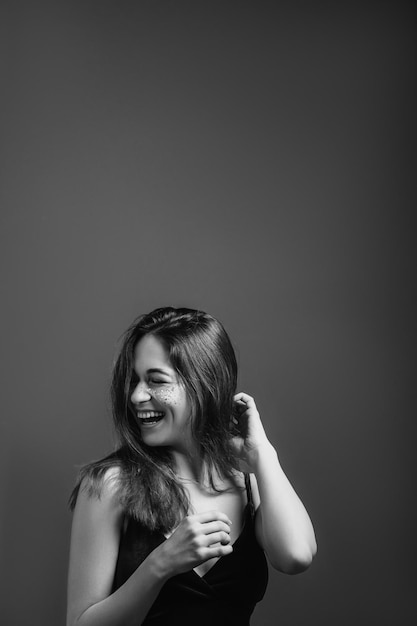In this classic black-and-white vertical portrait, a woman with medium-long, light brown hair parted down the center is caught mid-laugh. Her left arm is bent, with her fingers running through her hair, while her other arm is bent in front of her chest. She wears a thin-strapped black dress or top, which, along with her fair skin, stands out prominently against the very dark gray background. The woman’s body is facing slightly towards the camera but her head is turned to the side, laughing openly as if amused by someone or something off-frame. This candid moment is accentuated by the playful sparkles or glitter on her cheek, adding a hint of charm and flirtation to her infectious smile.